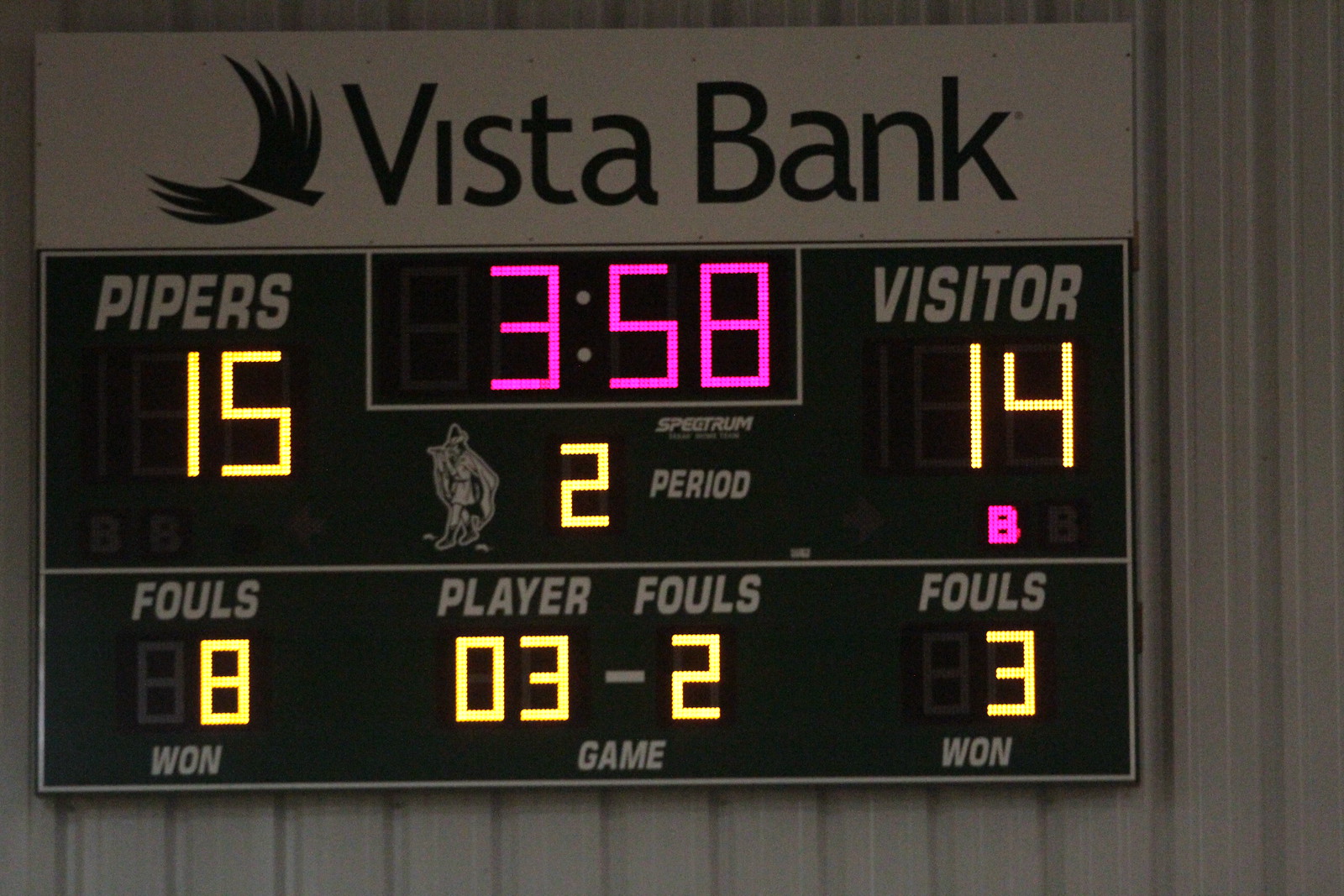This image captures a detailed view of a black scoreboard, prominently sponsored by Vista Bank, whose logo and name are displayed at the top against a white background. The scoreboard depicts a basketball game between the Pipers and a visiting team. The Pipers' current score is 15, highlighted in yellow letters, while the Visitors' score is 14, also shown in yellow. A digital clock centered on the scoreboard, illuminated with pink numbers, indicates there are 3 minutes and 58 seconds remaining in the second period. Below the clock, the fouls information is presented in white and yellow text against a black background. Specifically, it states there are a total of eight fouls, with the Pipers' players having accumulated fouls denoted as three players with two fouls and three fouls respectively. The scoreboard is mounted on a gray slate-colored wall, adding to the vivid and organized visual layout.